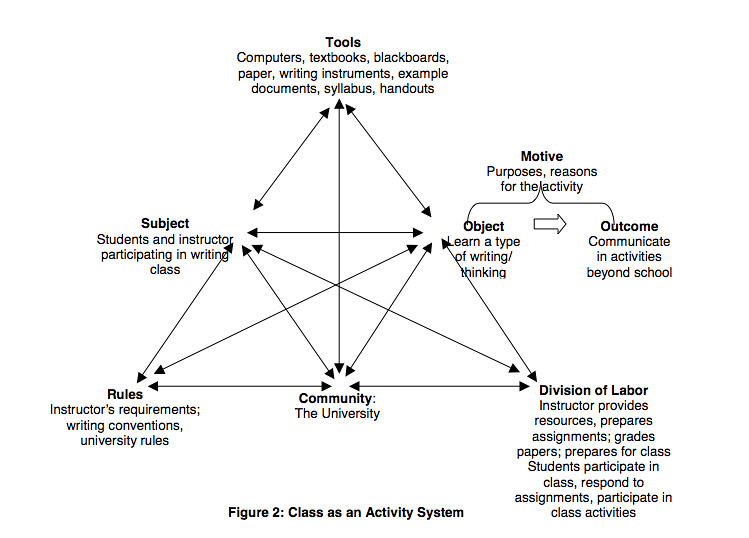The image is a detailed diagram on a white background with black text, structured around an inner and outer triangle, connected by various arrows. At the top, the heading "Tools" is followed by specifics such as computers, textbooks, blackboards, paper, writing instruments, example documents, syllabus, and handouts. The left section is labeled "Subjects," identifying students and instructors participating in a writing class. Below that, "Rules" lists instructional requirements, writing conventions, and university rules. The central part, marked "Community," denotes the university. Adjacent to this is "Division of Labor," detailing roles such as instructors providing resources, preparing assignments, grading papers, and students participating in class activities. At the right side, "Object" aims to teach a type of writing or thinking, connecting to "Motive," which addresses the purposes and reasons for the activity, and leads to "Outcome," which focuses on communication and activities beyond school. The diagram, captioned as "Figure 2: Class as an Activity System," uses arrows to illustrate the complex interactions within this educational framework.